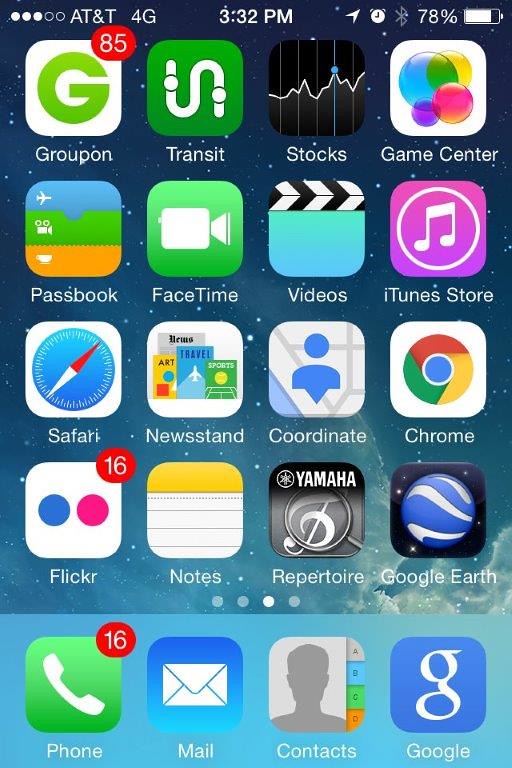The image depicts a smartphone screen with a detailed layout of apps and icons. At the top of the screen, cellular network bars are displayed showing three out of five bars, indicating a connection with AT&T and 4G service. The current time, 3:32 PM, is centrally located, flanked by icons for an arrow, an alarm clock, and an unlit Bluetooth logo, alongside a battery icon showing 78% charge.

The bottom dock contains four primary app icons: 'Phone' with 16 notifications as indicated by a red circle in its top right corner, 'Mail,' 'Contacts,' and 'Google,' each represented with its respective icon. The main portion of the screen shows a grid of 16 apps arranged in a 4x4 configuration, and it appears to be on the third page of the app list, as denoted by the third of four dots being highlighted.

In the top-left corner of the grid, there is the 'Groupon' app, which has 85 notifications. Following it are 'Transit,' 'Stocks,' and 'Game Center.' The second row hosts 'Passbook,' 'FaceTime,' 'Videos,' and 'iTunes Store.' The third row includes 'Safari,' 'Newsstand,' 'Coordinate,' and 'Chrome.' The fourth and final row features 'Flickr' with 16 notifications, 'Notes,' 'Repertoire,' and 'Google Earth.' Each app is associated with its respective icon.

The background of the screen is a starry night sky with clouds at the bottom, adding a celestial vibe to the phone's interface.